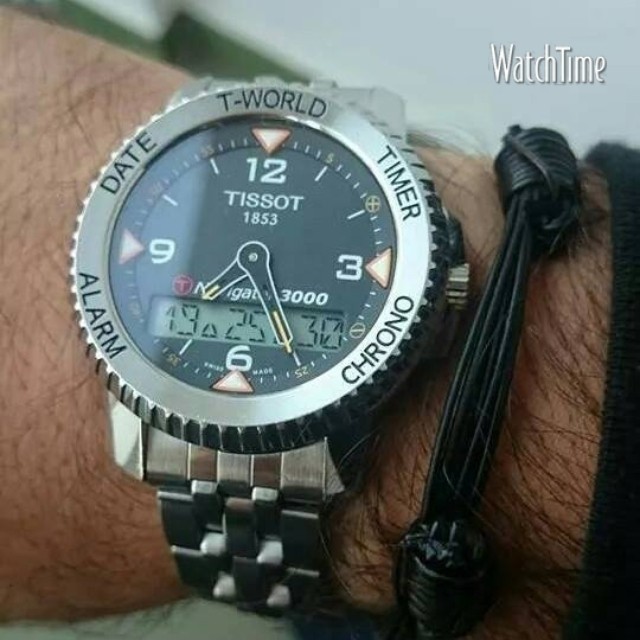The image is a realistic square photograph, predominantly featuring a light-skinned, black-haired wrist adorned with a stainless steel Tissot watch. The light gray background in the top right corner displays the text "Watch Time" in white font with a black shadow, giving a watermarked appearance. The central focus is on a man's wrist, which is also wearing a black leather wristband and is dressed in a black sleeve.

The Tissot watch features a stainless steel band and edge. The black watch face is marked with four orange-edged triangles at the 12, 3, 6, and 9 positions, while the numbers themselves are in white. The other hour markers are designated by dashes. The watch displays both analog and digital time, with the brand name "Tissot 1853" emblazoned in white text on the face. The analog clock shows the big hand pointing towards 5 and the small hand between 7 and 8. Surrounding the watch face are inscriptions in black text indicating "T-World, timer, chrono, alarm, and date," hinting at its multifunctional capabilities. The image likely serves as a sophisticated advertisement for the Tissot Navigate 3000 model watch.